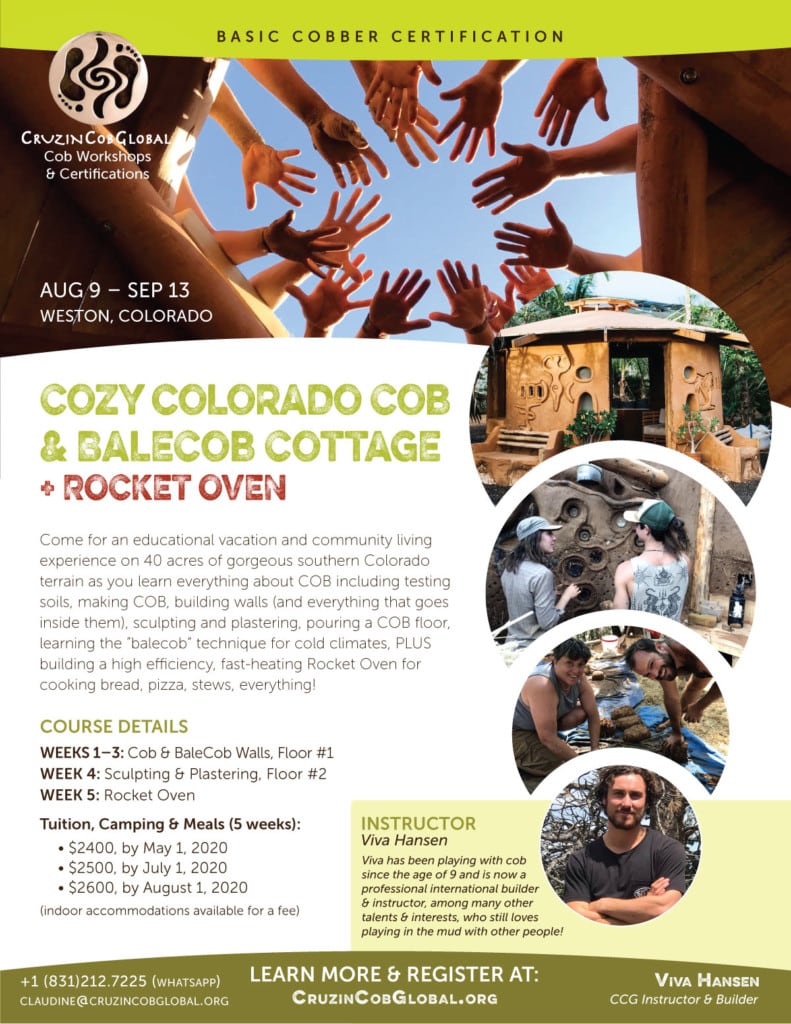This comprehensive flyer advertises the Cozy Colorado Cob and Bale Cob Cottage and Rocket Oven Basic Cobber Certification, promoting an educational vacation and community living experience. The certification course, running from August 9th to September 13th, will be held on 40 acres of beautiful Southern Colorado terrain. It promises to teach participants everything about cob construction, including testing soils, making cob, building walls, sculpting and plastering, pouring a cob floor, and mastering the bale cob technique for cold, wet climates. The course also includes building a high-efficiency, fast-heating rocket oven suitable for cooking a variety of foods. 

Detailed course breakdown:
- Weeks 1-3: Cob and Bale Cob Walls, Floor 1
- Week 4: Sculpting and Plastering, Floor 2
- Week 5: Rocket Oven

Tuition rates are $2,400 by May 1st, 2020, $2,500 by July 1st, 2020, and $2,600 by August 1st, 2020. The flyer features various images, including participants building and working together, and the instructor, Viva Hansen, who has been involved with cob since the age of nine and is now a professional instructor and builder. Contact details for more information include Claudine at CruisingCobGlobal.org and the WhatsApp phone number 1-831-212-7225. At the top of the flyer, a heartwarming image of hands together in unity through a building’s roof hole exemplifies the community spirit of the course.